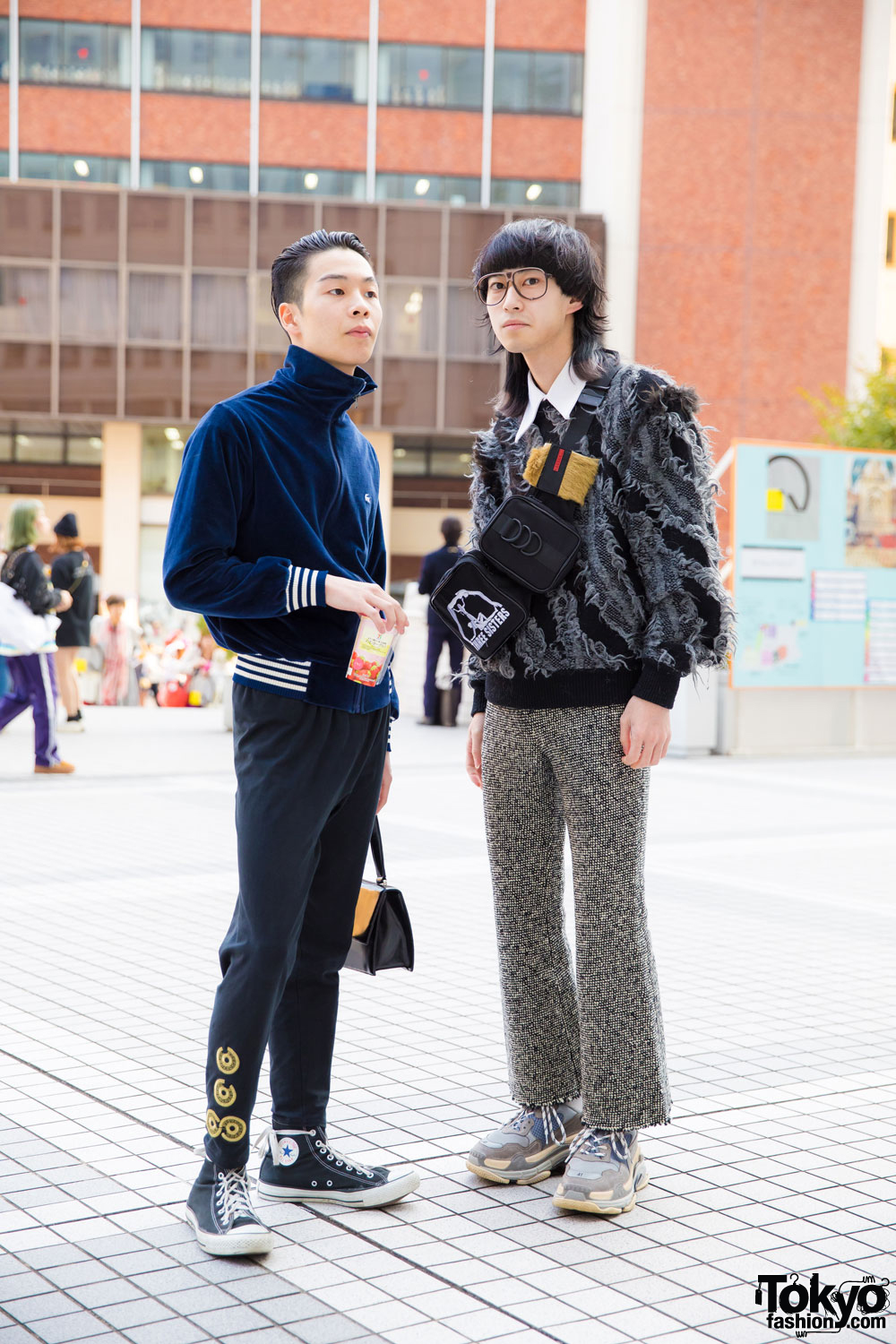The image captures two young Japanese men standing centrally in a tile-paved courtyard in front of a large red brick building, likely a university or government edifice. Both men, appearing to be in their early 20s, epitomize Tokyo street fashion. The man on the left is dressed in a vibrant blue velour tracksuit with white stripes along the sleeves and waist, complemented by black high-top Converse sneakers. He holds a purse in his left hand and a white plastic drink cup with a red bottom in his right. His dark black hair is styled neatly, and gold round symbols embellish his pants at the ankles. The man on the right showcases a more layered look with a distressed gray and black puffy jacket over a white shirt, paired with heavy black and gray woolen houndstooth-patterned pants and gray running shoes. His longer black hair and large glasses complete his ensemble, along with a backpack slung over his front. Both men are looking directly at the camera, exuding confidence and contemporary urban style. In the lower right corner of the photograph, the text "TokyoFashion.com" anchors the scene to the vibrant Tokyo fashion landscape.